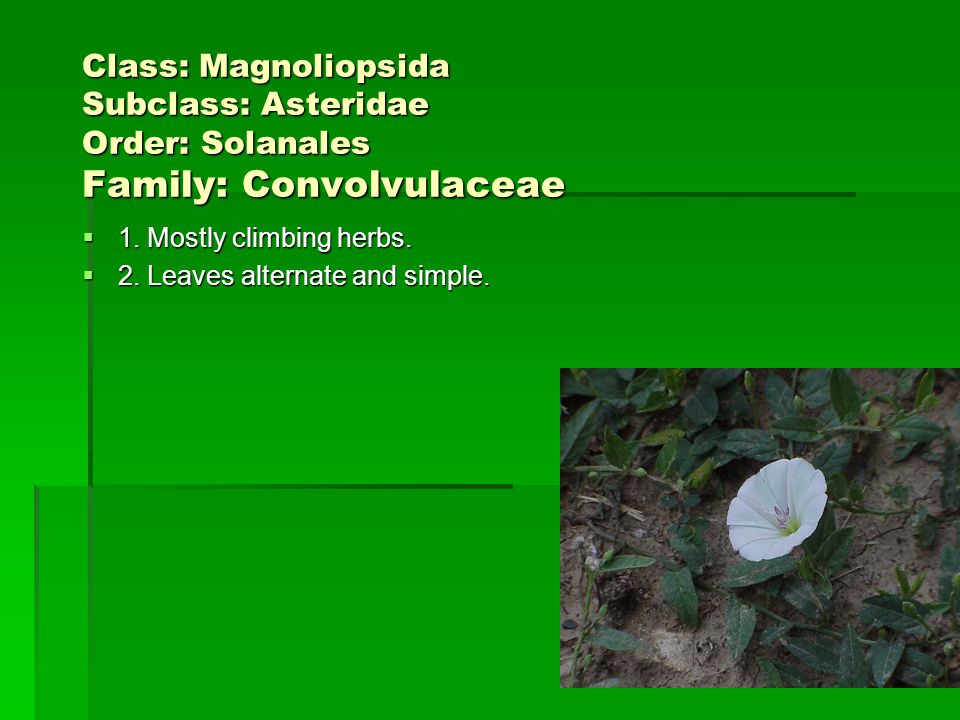The image is a dark green slide resembling a presentation, featuring a detailed botanical description. In the top left corner, the text in creamy white font is organized into four lines, stating: "Class: Magnoliopsida," "Subclass: Asteridae," "Order: Solanales," and "Family: Convolvulaceae." Below this classification, two bullet-pointed characteristics of the plant are listed: "1. Mostly climbing herbs," and "2. Leaves alternate and simple." The bottom right corner of the image captures a white flower with a pink center, surrounded by green leaves growing out of the dirt floor. The flower, reminiscent of a horn from an old-style record player, is clearly defined against the dark green backdrop with minimal right-angled lines.